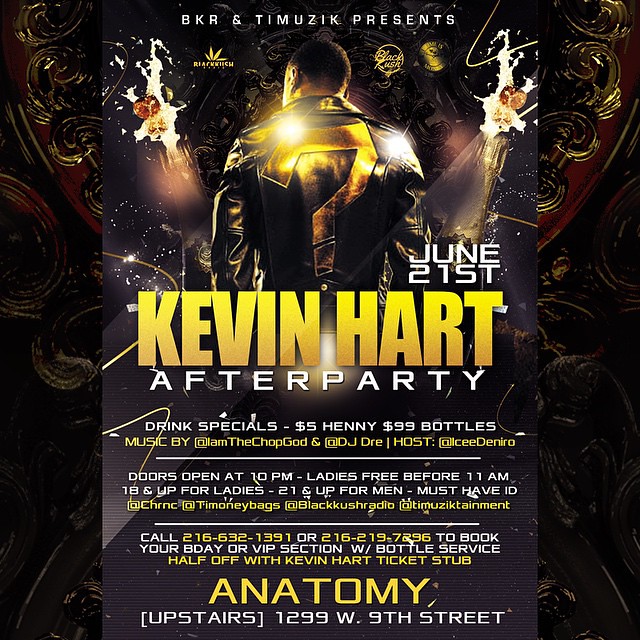The image depicts a promotional poster for a Kevin Hart after-party event, prominently featuring the following details. Centered on the mostly dark and textured background, the poster announces "BKR and T-Music Presents Kevin Hart After-Party" with "Kevin Hart" in bold gold text and "after-party" in white beneath it. The event takes place on June 21st. A photograph of Kevin Hart, seen from the back in a black leather jacket adorned with a gold question mark, is also displayed. The poster specifies drink specials, including $5.00 honey and $99.00 bottles, with music by I Am The Chop God and DJ Dre, and hosted by Ice Deniro. It mentions that doors open at 10 p.m., with ladies gaining free entry before 11 a.m. Entry requirements are 18 and over for ladies and 21 and over for men, with mandatory ID checks. At the bottom, in gold text, it notes the event location "Anatomy" on "Upstairs 1299 West 9th Street" and includes contact information for booking and VIP section service, offering half-off bottle service with a Kevin Hart ticket stub.